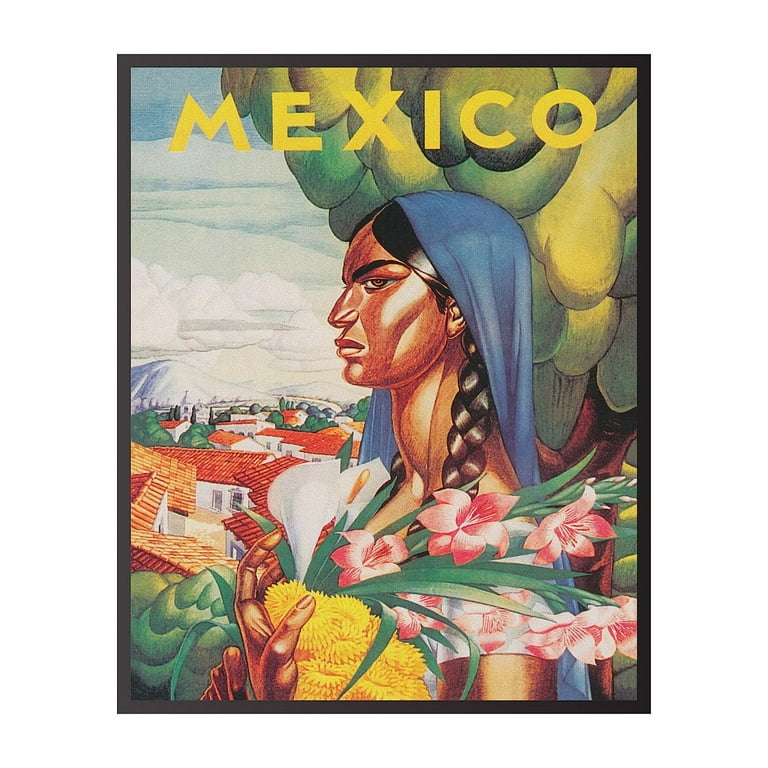This vibrant illustration, reminiscent of a travel poster, prominently features the word "Mexico" in bold yellow text at the top. Dominating the image is a Mexican native woman with braided black hair flanking either side of her neck. She dons a blue headscarf that drapes down elegantly. Her skin is a warm bronze tone, highlighting her strong facial features. Cradling her armful of bright yellow, pink, and white flowers accented with greenery, she exudes a serene presence. In the background, to the left, lies a picturesque small Mexican town with white buildings capped with orange terracotta rooftops. Further beyond the town, fields stretch out towards majestic white mountains under a cloudy sky, all bathed in a colorful and inviting palette intended to inspire travel to Mexico.